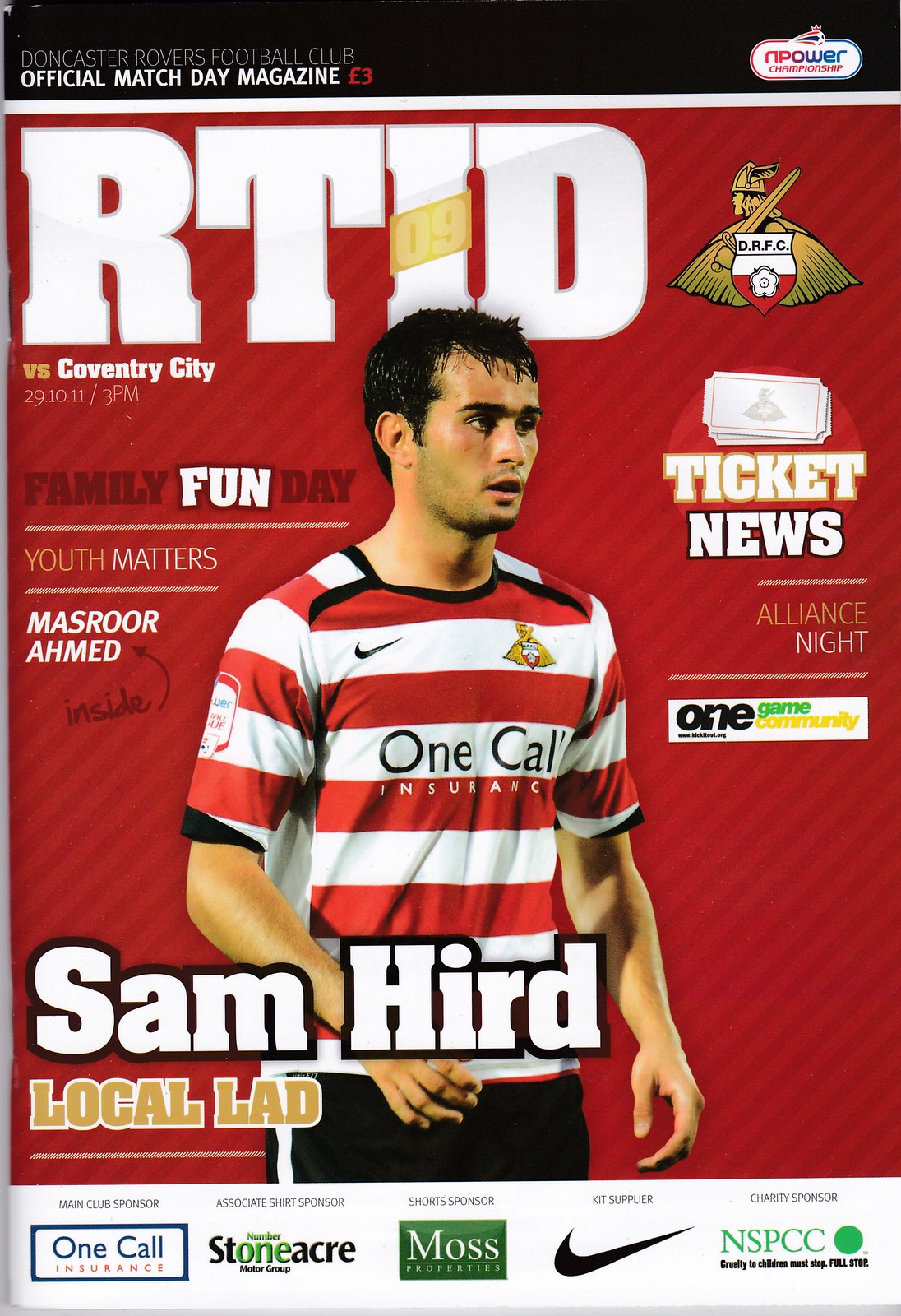The image is the cover of a Doncaster Rovers Football Club Official Match Day Magazine, priced at three British pounds. It features a young Hispanic man with short, shiny black hair, a clean-shaven face, and intense brown eyes. His face is slightly red and sweaty, indicating the photo was taken during a game. He is wearing a red and white striped jersey with the text "One Call Insurance" across his chest, a Nike insignia on the left, and another emblem on the right. Above him, the magazine title "RTID" has a yellow banner with "09" over the letter "I". Below, sections titled "Versus Coventry City," "Family Funday," "Youth Matters," and "Masoor Ahmed" are mentioned. The name "Sam Hurd" is prominently displayed across his image, labeled as "Local Lad". The background of the cover is patterned with red and dark red stripes, and it includes various sections like "Ticket News" and "Alliance Night". A series of sponsors, including Nike, One Call Insurance, Stoneacre Motor Group, Moss Properties, and NSPCC, are listed at the bottom. The club's logo, a Viking holding a sword in front of a shield with "DRFC" and red accents, is present as well.